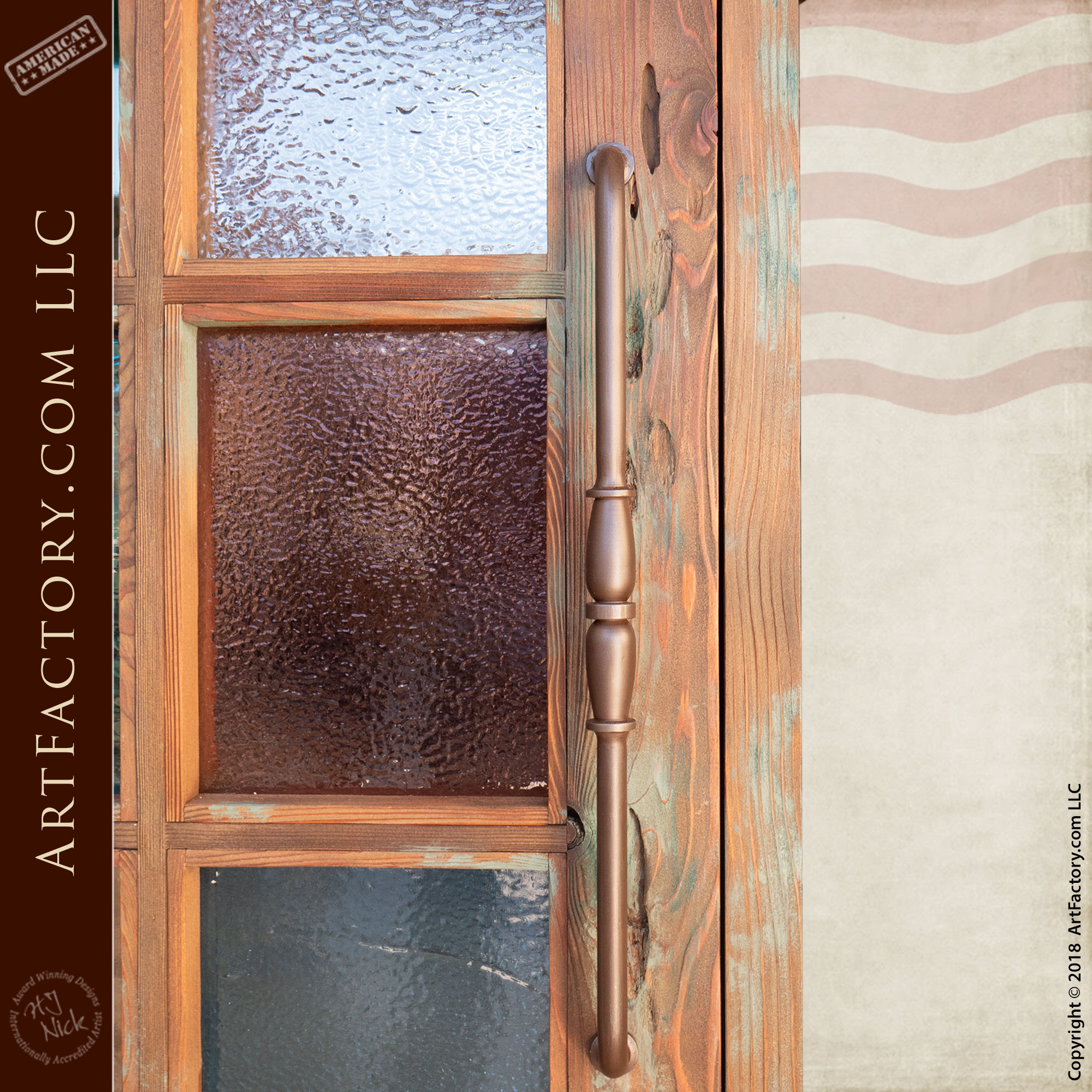The image from artfactory.com LLC, copyrighted in 2018, depicts a meticulously crafted wooden door made of solid oak. Prominently featured is a long, intricately designed brass door handle, adding an artistic flair. The door incorporates multiple small panes of stained glass—each in muted hues of blue, maroon, and clear—though frosted enough to obscure visibility, ensuring privacy. The glass panes are simply colored, devoid of additional decorative elements. To the left, a vertically placed banner bears the artfactory.com LLC name, and at the top, a logo states "American-Made" with additional text about award-winning craftsmanship by H.J. Nick. The surrounding door frame is also wooden, blending seamlessly into a slightly decorated wall, which exhibits a subtle wave-like paint design in the upper right-hand corner of the image.